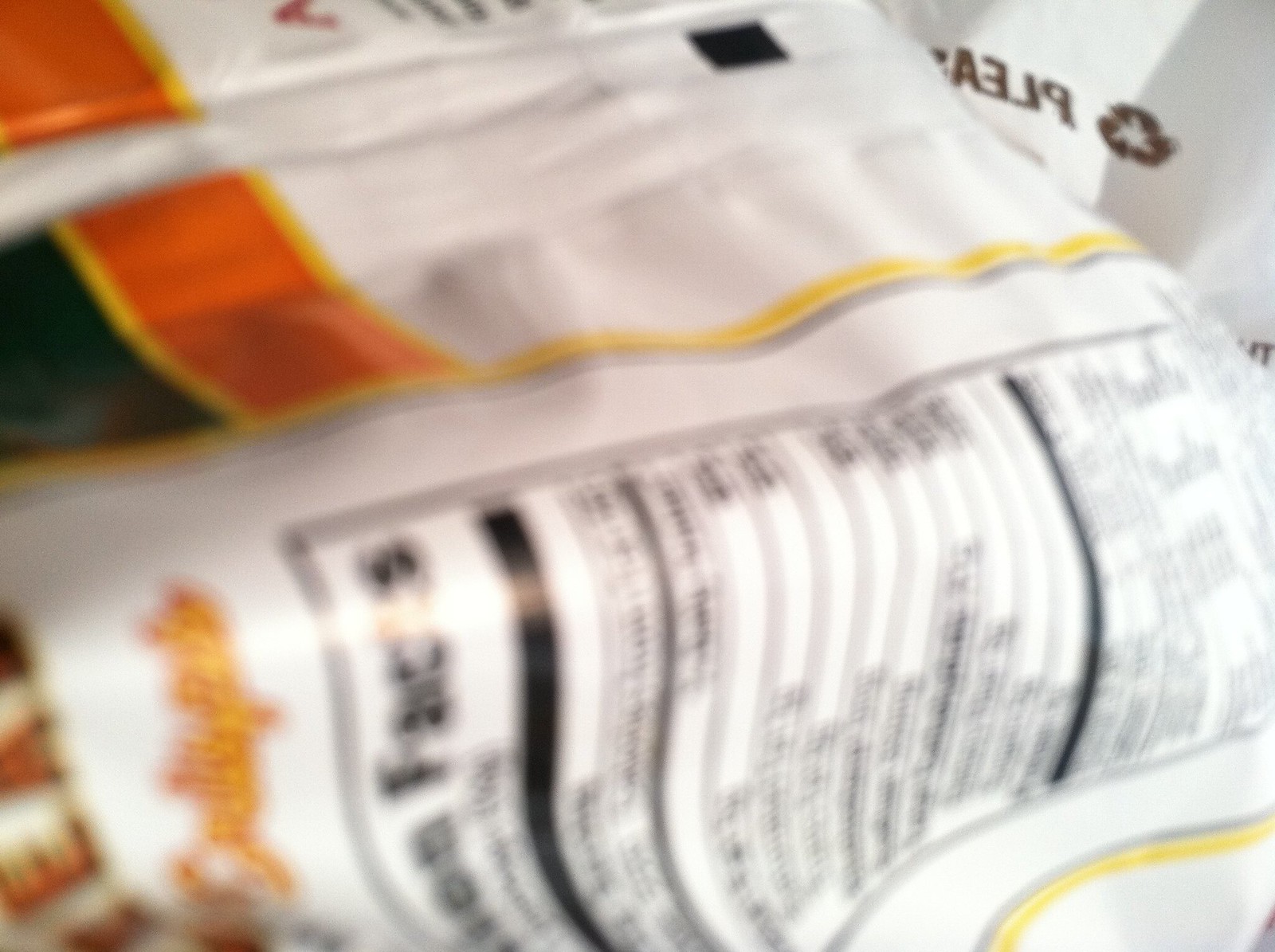The image shows a blurry close-up of a horizontal or landscape-oriented Peppa Pig food container that is lying sideways on a table. The predominantly white plastic packaging features colorful designs in red, green, yellow, and black. Notably, a black and orange logo can be seen amidst the design. A detailed nutritional facts table, written in black, runs from top to bottom, accompanied by a recycling logo in the top right corner, also in black with the word "please." Some gold colors appear in the bottom left of the image. The overall image is unfocused, making specific text difficult to read, but the vibrant, mixed colors and clear nutritional facts mark its significance.